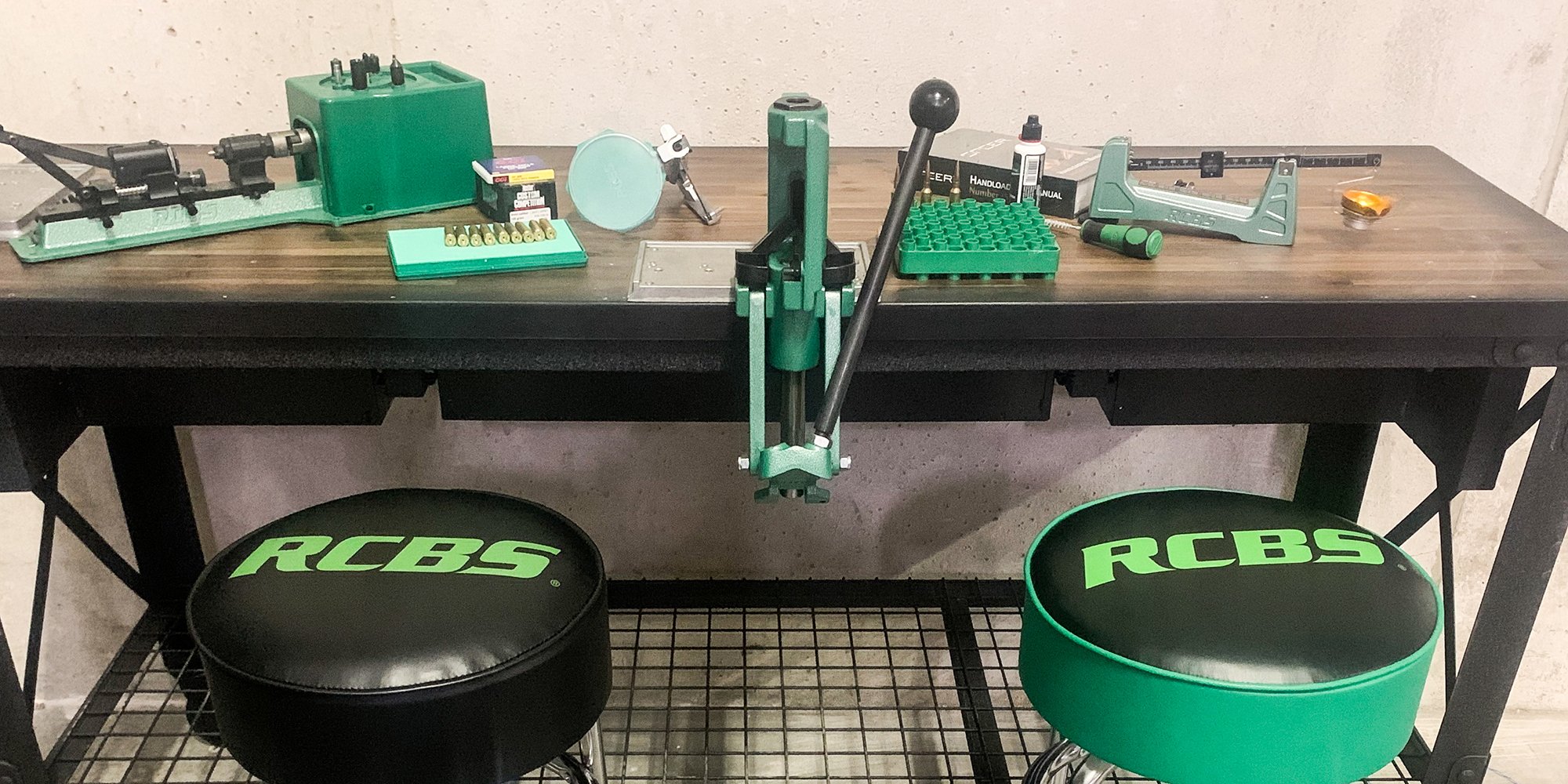The photograph captures a robust brown wooden table with sturdy black metal legs, set against a light pink or white background. The tabletop is scattered with various specialized tools, prominently green and some gold, indicating a workspace likely dedicated to machining or reloading. Central to the setup is a black spool connected to a black metal arm, which is in turn attached to a green box. Additionally, a green clamp or arm extends from the middle, culminating in a long black handle with a black bulb at the end. Nearby, smaller measuring tools, including a screwdriver, are also visible. Surrounding the table are two backless stools with cushion tops and mesh flooring beneath. The stool on the left features a black leather cushion with the brand "RCBS" in green, while the stool on the right has a green cushion with "RCBS" inscribed in black. This detailed and organized setup hints at a dedicated and professional workspace for precise technical work, possibly involving the reloading of bullets, with green holders and small gold tablets that resemble bullet components.